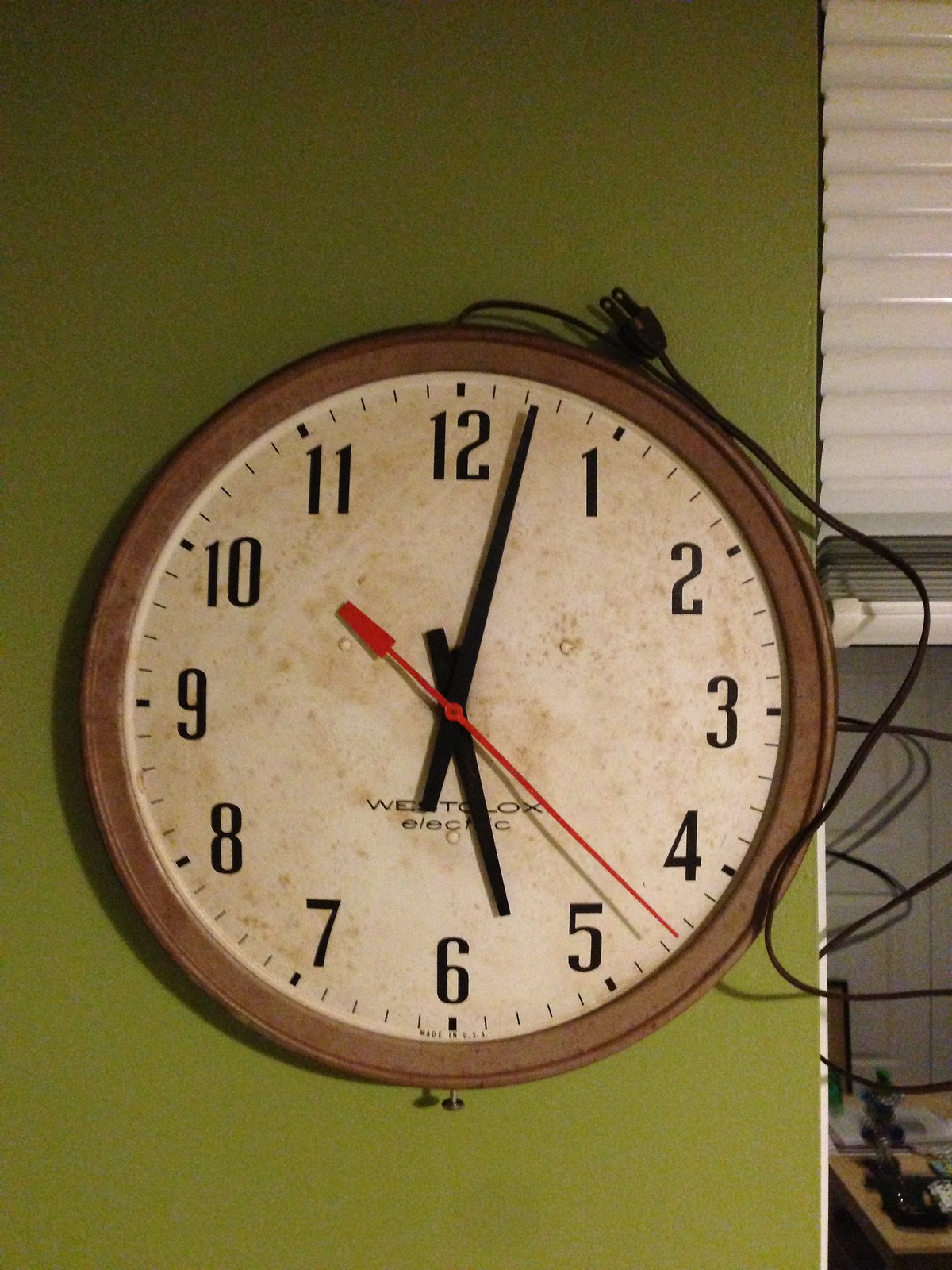The photograph depicts a vintage analog clock mounted on a green wall. The clock features a round, wood-toned frame with an off-white interior that appears aged or musty. Black numbers, 1 through 12, are clearly marked on the clock's face with small dashes in between to indicate minutes. The clock's hands include a large black minute hand positioned between the 12 and the 1, a shorter black hour hand between the 5 and the 6, and a slender red second hand between the 4 and the 5, showing the time as 5:03. A black electrical cord drapes across the top of the clock, hanging down to the bottom but not plugged in. To the right of the clock, there are white plastic mini blinds covering a window, and below the blinds is a section of gray tiled backsplash, suggesting the location might be a kitchen.